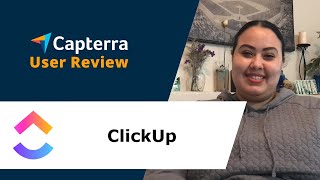A screenshot of the Capterra User Review website is depicted. On the left side of the screenshot is the word "Capterra" in white text, positioned above a line of text reading "User Review" in yellow. Adjacent to "Capterra" is an arrowhead design that is split into two colors: teal on the top half and orange on the bottom half. To the right of the text, the background transitions from a dark green to an image of a woman smiling in a living room. She is dressed in a grey hoodie with her hair pulled back and stands in front of a fireplace. A white banner occupies the lower half of the page, displaying the word "ClickUp" in black text without any spaces. Positioned to the left of the "ClickUp" text is the company's rainbow-colored logo.